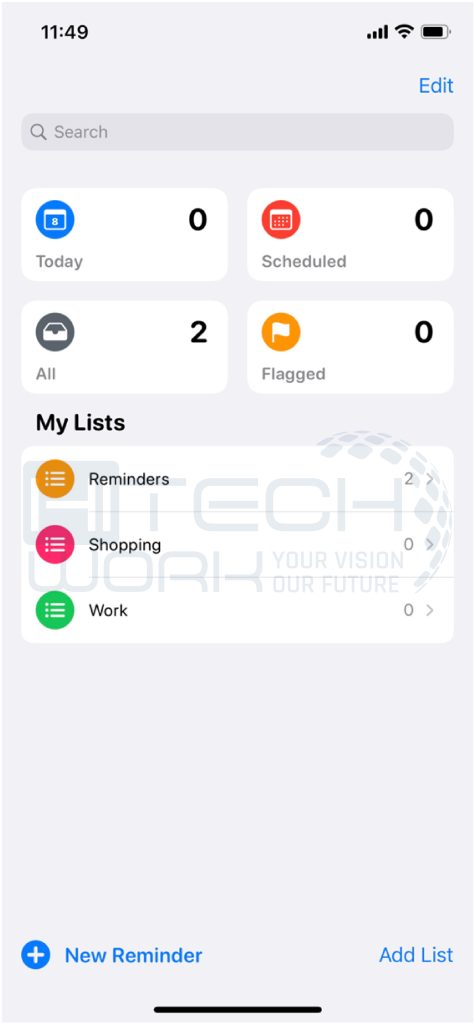The image is a detailed screenshot from a cell phone, set against a gray background. The timestamp "1149" appears in black text at the upper-left corner. At the upper-right corner, contact icons are displayed: all cell reception bars are fully lit, the Wi-Fi icon is visible, and the battery icon shows a full charge. Beneath the battery icon, "EDIT" is written in blue text, followed by a gray search bar featuring a magnifying glass icon and the word "SEARCH."

Below, in the main area, two white boxes are positioned side by side. The left box features a blue circle with the word "TODAY" above a bold number "0". The right box shows a red circle with a calendar icon above the word "SCHEDULED" and another bold "0". 

Further down, additional boxes appear: on the left is an icon resembling a filing cabinet with the word "ALL" next to the number "2." To the right, an orange circle with a white flag icon is next to the word "FLAGGED" and another bold "0". 

In the lower section, against the gray background in black text, the heading "MY LISTS" is prominently displayed, followed by a list of items: "REMINDERS," "SHOPPING," and "WORK."